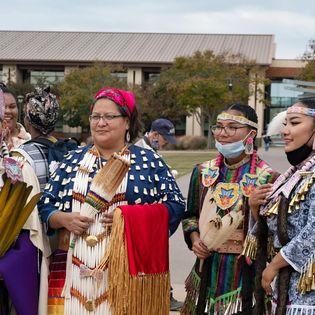This image features a group of predominantly Native American women, all dressed in vibrant traditional attire adorned with intricate beadwork and fringes. Central to the scene is a woman wearing a blue top with white spots and a beaded necklace cascading down the front of her dress. She holds a multi-colored whisk-like device featuring hues of brown, white, purple, yellow, and green. Draped over her left arm is a straw blanket with brown fringe, and she’s accessorized with a pink scarf in her hair.

To her right, two more women in equally colorful Native dress can be seen. One is clad in a multicolored top with fringes and has a feather arrangement in her hands, complemented by a blue mask and a headband. The other woman wears a blue-and-white top with a matching headband and features a scarf with tassels around her neck. Surrounding them, other women in traditional dress are engaged in conversation, smiling and appearing to be in good spirits.

In the background, a man wearing a blue cap and mask is visible but does not appear to be part of the main group. The photograph captures a moment of cultural pride and community, showcasing the rich heritage and varying ages of the participants.